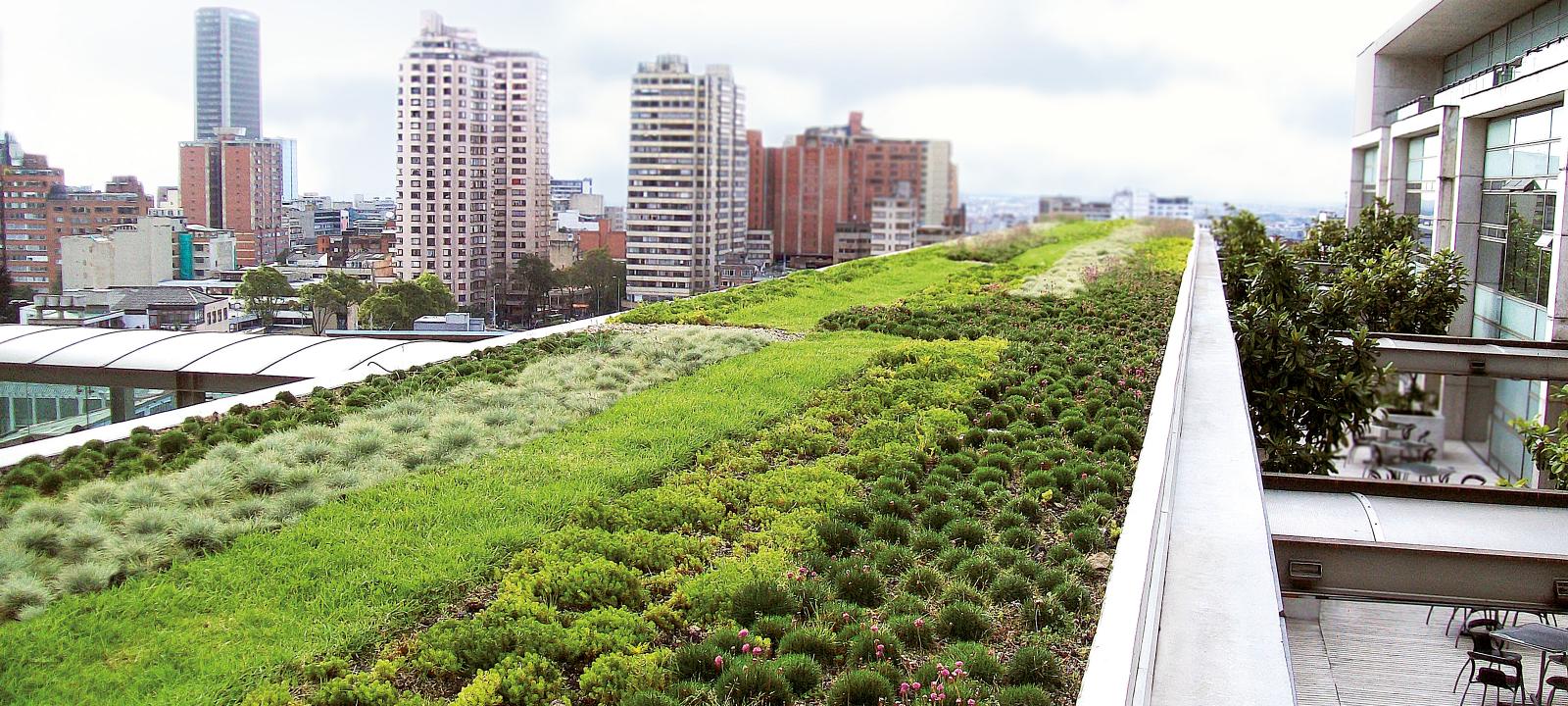This detailed outdoor photograph captures a vibrant rooftop garden spanning from the bottom left corner to the far edge of the image. The roof, transformed into a lush green space, features bands of spiky green plants, dense patches of grassy areas, and more spiky vegetation, embodying the modern trend of converting rooftops into eco-friendly green spaces that provide food and oxygen. 

To the right of this elevated garden, a walkway with black tables and chairs is set in front of a sleek glass and steel building. On the left side of the image, the city skyline is visible, showcasing a mix of brick buildings, high-rises, and a particularly tall skyscraper. The sky above is a blend of gray and blue, adding a touch of haze to the urban landscape. 

Overall, the photograph is rectangular and horizontal, emphasizing the expansive green rooftop against the urban backdrop, with no readable text present.